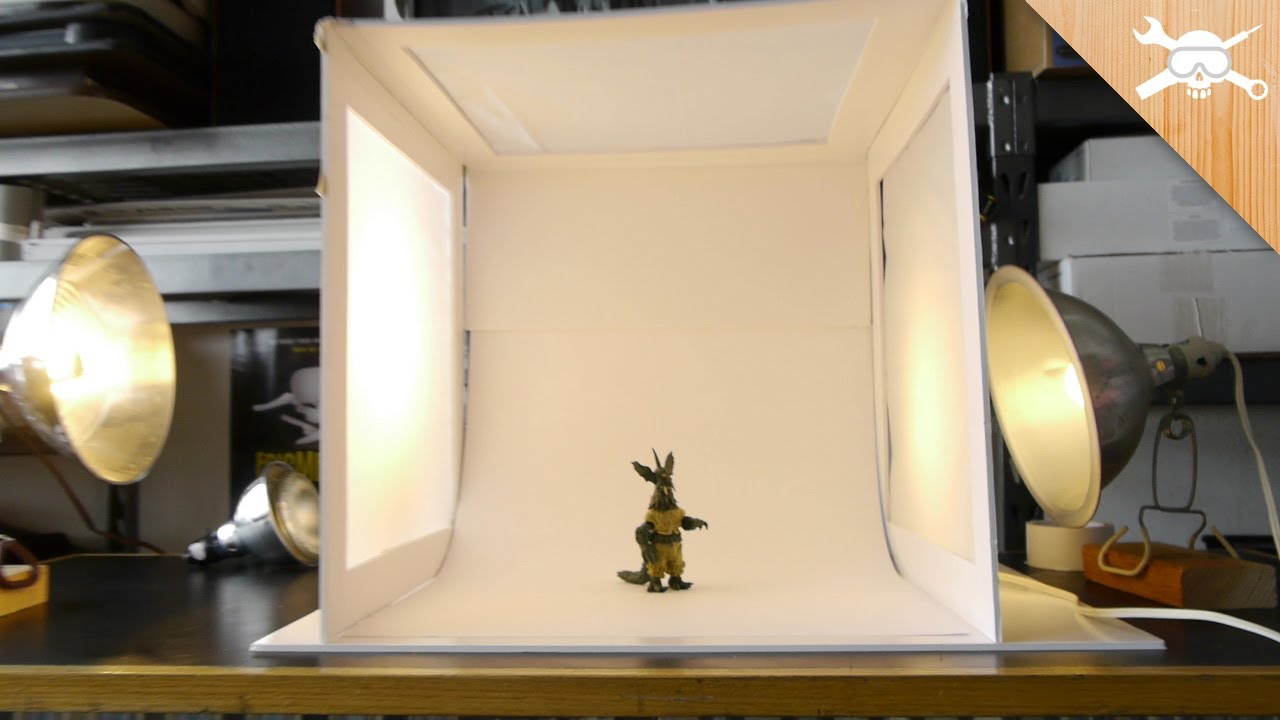The image depicts a detailed studio setup for potentially creating stop-motion animation or capturing promotional shots. At the center of the setup is a white light box with semi-transparent paper sides, designed to diffuse the illumination provided by the studio lights positioned on either side of the box. These lights are perfectly directed to shine through the paper, creating a soft and even light inside the box.

Inside the light box stands a detailed figurine of an anthropomorphic creature, appearing to be a mix between a lizard and a furry monster. This character has striking features such as long pointy ears and a long tail, and it is dressed in clothes that resemble a yellow or tan military jumpsuit, adding a distinct personality to the figure. The creature's fur is described as either brownish or black.

The entire setup rests on a wooden desk amidst a cluttered background that includes other studio equipment, white boxes, and wires, suggesting a busy workspace. There is also a noticeable logo in the top right corner of the image, which features a skull wearing safety goggles over a crossed wrench and a soldering iron, adding to the industrial and creative atmosphere of the setting.